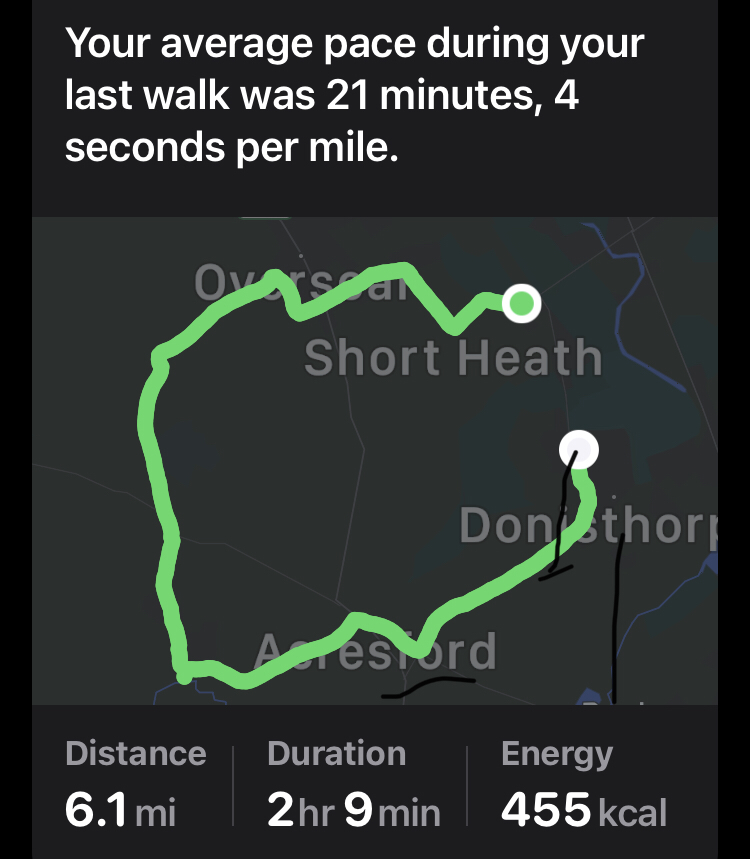The image is a nearly square, portrait-oriented screenshot from a fitness tracking app, possibly Fitbit. The background is predominantly black, enhancing the visibility of the various informational elements. At the top, a gray rectangular bar contains white text that reads: “Your average pace during your last walk was 21 minutes, 4 seconds per mile,” spread over three lines.

Beneath this bar, a dark gray, GPS-based map shows a trail. This map is accentuated by thick green lines forming an almost looping path. The starting point of the trail is marked by a white circle with a green dot inside, while the ending point is marked by a plain white circle. Along the trail, certain locations are identified in light gray text, including “Short Heath” and “Donnesthorpe,” though the green trail partially obscures some names.

At the bottom of the image, a gray bar provides further statistical details in white bolded text: on the left, "Distance" with a record of 6.1 miles; in the center, "Duration" showing 2 hours and 9 minutes; and on the right, "Energy" displaying 455 kcal. The detailed representation and style suggest that this is a fitness tracking screenshot designed for close monitoring of physical activity.